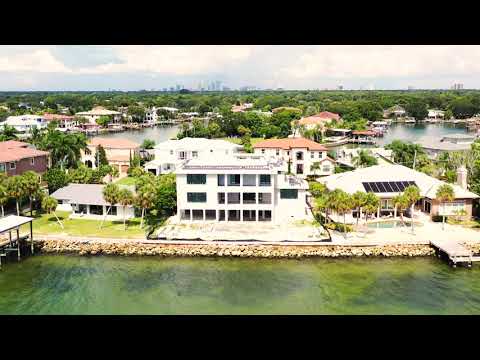The image depicts a picturesque waterfront community, likely a luxurious enclave or a retirement area. Dominating the foreground are clear, green-tinted waters framed by rocky shores and scattered docks. The centerpiece is a striking, three-story modern home with abundant windows, and an open ground level, presumably for storing water sports equipment. Adjacent to it, another significant house features solar panels and a dock. The scene is dotted with multiple homes, varying in design from white facades with reddish roofs to other distinctive structures, all nestled among lush trees. The background reveals a cloudy sky, though the sun illuminates the entire area, casting a bright, welcoming light over the waterfront properties. The overall vibe resembles a high-end resort or a serene peninsula, with homes seamlessly integrated into the natural landscape.